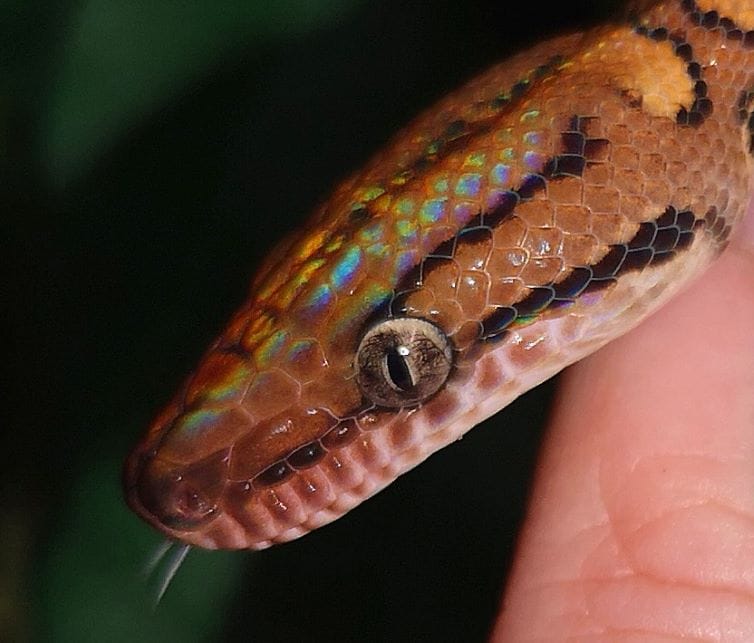The photograph depicts a vivid, up-close profile of a small, live snake's head, angled downward and to the left. The snake's head, captured just before its neck begins, reveals intricate details including its gray, forked tongue darting out with a slight motion blur, indicative of a recent lick. Its eye, featuring a vertical slit pupil, is a blend of gray, brown, beige, and black hues. Below the eye, the snake's lower jaw exhibits a creamy gray tone, transitioning into white scales around its mouth. Above this, a striking dark brown stripe runs up toward the nose, complemented by another stripe extending from the eye.

Reflecting the light, the scales atop the snake's head display an iridescent sheen, casting hues of green, yellow, and blue, enhancing its mesmerizing appearance. The snake's body continues with swirling dark brown markings interspersed with an orange circle surrounded by a black line, though the image cuts off before showing more of its neck. The snake is held by a human hand, visible on the lower right, suggesting its small size. The background is a blend of light to dark green, creating a blurred, almost black backdrop that contrasts sharply with the snake's vivid colors.